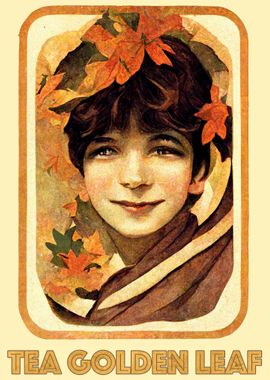This vintage-style advertisement for Tea Golden Leaf features a detailed illustration of a young Caucasian woman, likely in her early thirties, with a radiant smile. Set against a cream-colored background, the image is framed within a rounded rectangle. The woman has dark brown hair adorned with orange and yellow flowers, adding a vibrant touch to her appearance. She has light-colored eyes, is wearing makeup, and her complexion is fair. Her attire includes a brown shirt or shawl that covers her shoulders and most of her neck. Prominently displayed at the bottom of the advertisement, the text "Tea Golden Leaf" is written in light yellow and brown colors, reflecting a harmonious, vintage aesthetic.